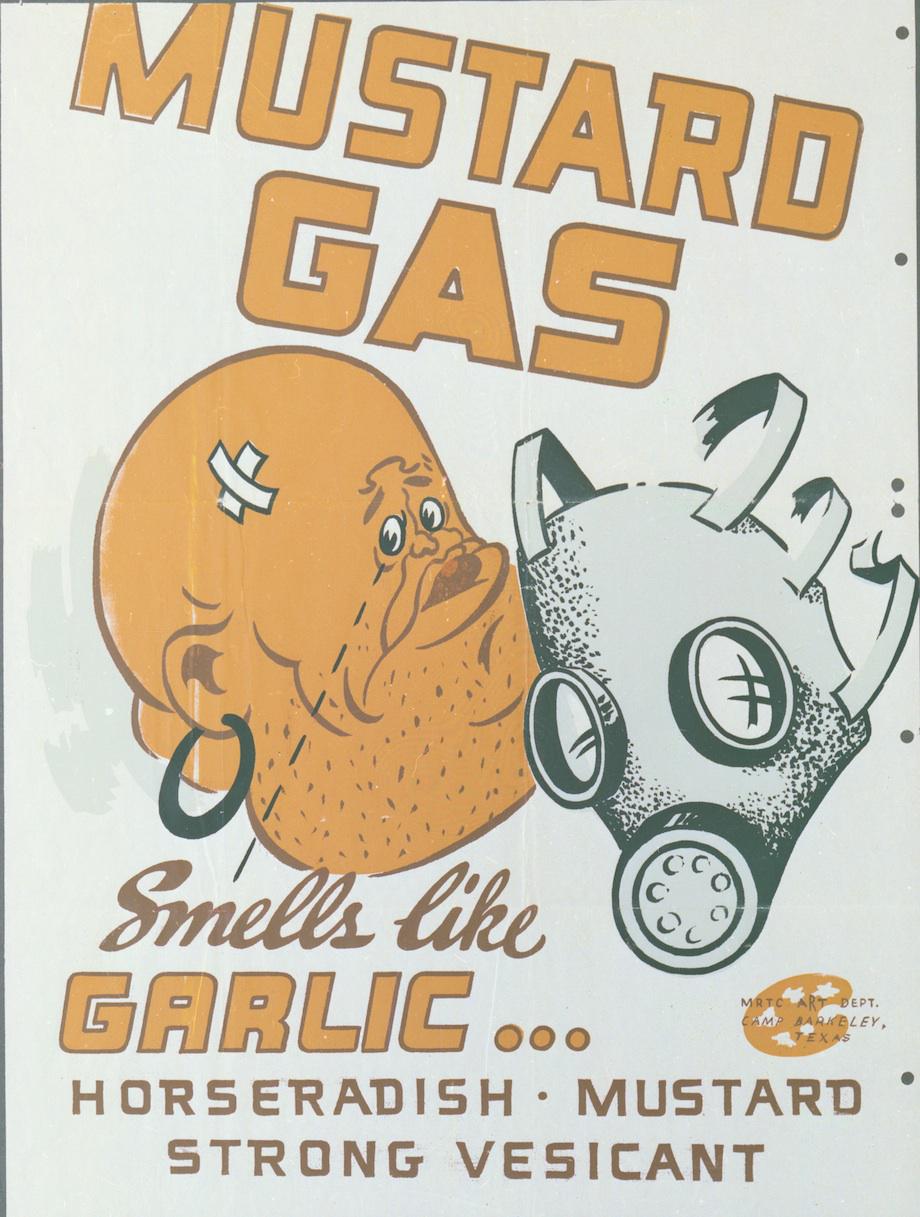The image is a vertical rectangular poster, likely from World War I. Dominating the upper left corner are the words "MUSTARD GAS" in bold, mustard-yellow letters slanting downward against a white background. Below this heading is an exaggerated depiction of a man's face in a side profile, with visible eyes, a small stubbly beard, and two criss-crossed white band-aids on his bald head. He wears a large black earring and has a sad expression. Adjacent to his face is an illustration of an old-time gas mask, reminiscent of those used in the world wars. Underneath the man's face, in cursive darker writing, it states "smells like," followed by "GARLIC" in large yellow letters. Below this, in darker text, it reads, "horseradish, mustard, strong vesicant." There is also a small logo or insignia representing the creator, possibly the MRTC Art Department, Camp Bengley, Texas. The poster's overall theme seems to depict the harsh and pungent nature of mustard gas, using striking visual and textual elements for emphasis.